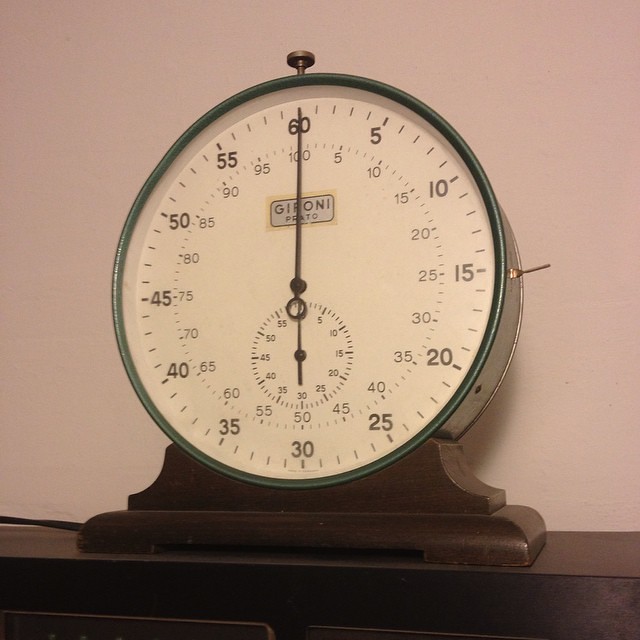This image depicts a vintage-looking timing device reminiscent of an old-fashioned alarm clock with an ivory face and brown numbers encased in a green metal frame. The clock face prominently displays a single black hand and a smaller section underneath for seconds. The numbers start at 60 at the top and increment by 5, moving clockwise around the face (5, 10, 15, etc.), with 30 at the bottom and 45 on the left, indicating its function as a timer rather than a traditional clock. At the top of the device is a black knob used to adjust the time, and the nameplate "Gironi" is visible at the center-top of the clock face. The timer is mounted on a substantial brown base, suggesting it is intended for use in a larger setting, such as a field. Additionally, a black cord extends from the device, indicating it can be powered through an electrical connection. The entire setup is positioned against a tan wall.